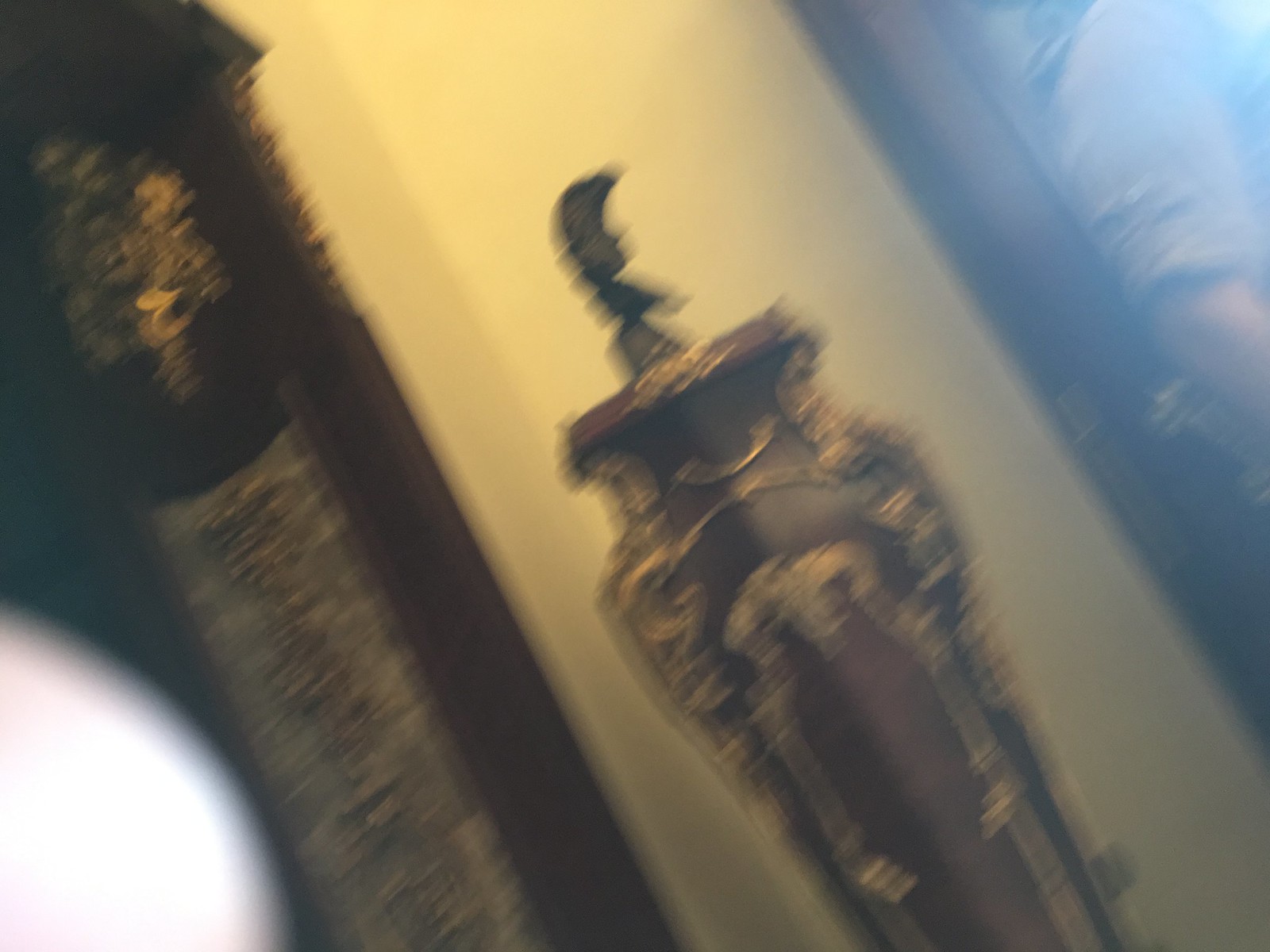This image, taken at a Dutch angle, features a very ornate and large vase or jar that appears quite old and possibly valuable. The vase, adorned with intricate gold lining and a detailed head profile of a man in a hat, suggests a significant artistic or historical value. The main colors of the vase seem to be gold and either maroon or dark wood. The photo is somewhat blurry, likely taken in a museum, antiquated house, or mansion, and might have been snapped hurriedly or secretly, as a finger is visible in the bottom-left corner, casting a white shadow. To the left of the vase, there appears to be a tall wooden casing, possibly a grandfather clock, with intricate gold details on its glass door. On the right, you can see a man's right arm in a rolled-up long-sleeved gray shirt against a background of various blurred colors, including blues and pinks. The wall in the background is a yellow-beige color, adding a muted backdrop to the detailed and vibrant objects.